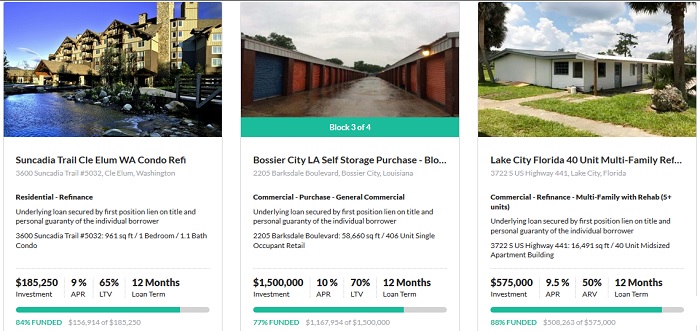This property listing site showcases three distinct investment opportunities, each represented by an image and detailed information banner.

1. **Sunkadia Trail, Washington Condo**
   - **Location:** Sunkadia Trail, COE, LM, WA (Washington)
   - **Price:** $185,250
   - **APR:** 9%
   - **LTV (Loan-to-Value):** 65%
   - **Loan Term:** 12 months
   - **Funding Status:** 84% funded
   - **Property Type:** Residential condo located by a river or lakefront
   - **Security:** Underlying loan secured by a first position lien on title and a personal guarantee from the individual borrower.

2. **Bossier Chili, Louisiana Self-Storage Facility**
   - **Location:** Bossier City, LA
   - **Price:** $1.5 million
   - **APR:** 10%
   - **LTV (Loan-to-Value):** 70%
   - **Loan Term:** 12 months
   - **Funding Status:** 77% funded
   - **Property Type:** Self-storage facility along a cement road with garage-style storage units in a single-level design.

3. **Lake City, Florida Multifamily Units**
   - **Location:** Lake City, FL
   - **Price:** $575,000
   - **APR:** 9.5%
   - **ARV (After Repair Value):** 50%
   - **Loan Term:** 12 months
   - **Funding Status:** 88% funded
   - **Property Type:** 40 unit multifamily complex.

These listings offer various real estate investment options with specific details on APR, funding status, and security measures, appealing to potential investors seeking residential, storage, or multifamily properties.